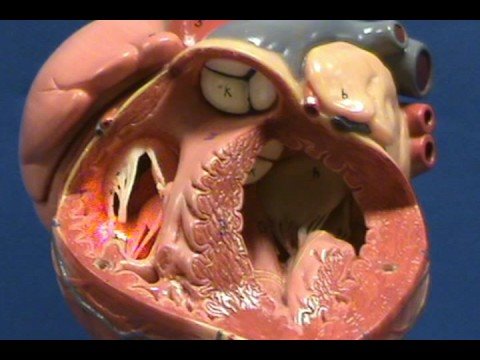The photograph depicts an intricate anatomical model of a human heart, showcasing a cross-section that reveals the detailed inner workings and structures. The model is labeled with letters, illustrating different components and valves. At the top left corner, a prominent pink section is visible, while the midsection displays various openings and cavities, including tricuspid valves and potentially other partially obscured valves. The model highlights the pulmonary artery and pulmonary vein, as well as distinct red veins and blue arteries that traverse the heart's surface.

In the foreground, the heart's interior is shown, with the surface revealing closed heart tissue and deeper layers exposing the muscle wall's varying thicknesses. The inside of the heart is characterized by spongy material lining the cavities, most notably seen in the large cavity on the right. The color scheme primarily comprises pink, white, blue, and red, with three tumorous white structures marked by a black letter "A" in the top cavity. There are also small connectors resembling tendons across the upper atrium, while the ventricle areas are less detailed, showing only the muscular inner formations. Overall, the model provides a comprehensive view of the heart’s anatomy, emphasizing the valves, cavities, and arterial structures.